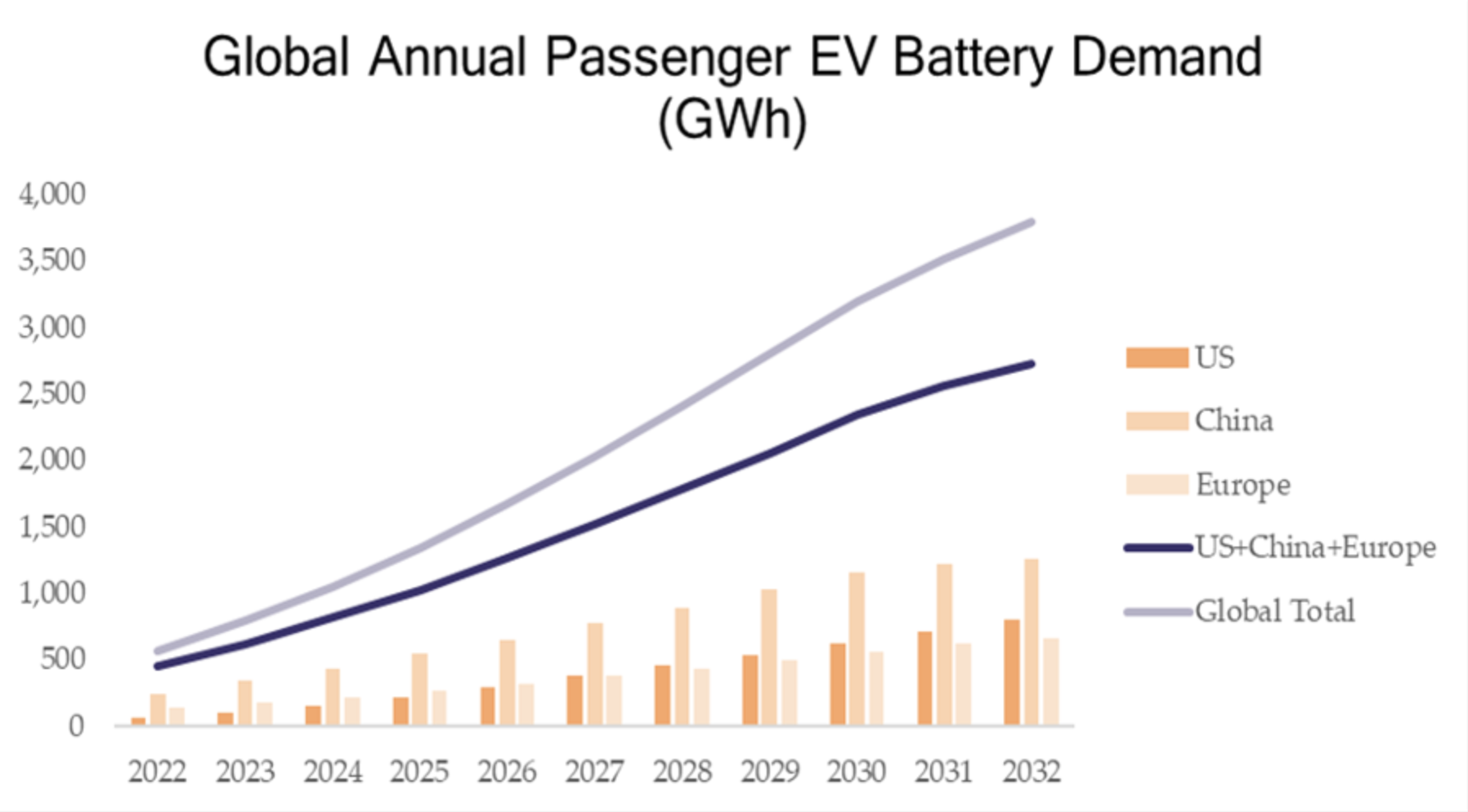The image depicts a detailed line graph with a bar chart superimposed, set against a white background. At the top in black text, it is titled "Global Annual Passenger EV Battery Demand (GWh)." The horizontal axis charts the years from 2022 to 2032, while the vertical axis ranges from 0 to 4000 GWh. The right side features a legend that identifies various color codes: orange bars indicate the U.S., light peach bars indicate China, and light pink bars indicate Europe. Additionally, there are lines representing cumulative data: a dark blue line for the combined demand of the U.S., China, and Europe, and a light purple line for the global total. 

The bar chart below shows demand trends for each region from 2022 to 2032. China's demand consistently ranks the highest, followed by relatively similar demands from the U.S. and Europe. The combined demand for the U.S., China, and Europe rises from 500 GWh in 2022 to approximately 2500 GWh in 2032. The global total increases from 500 GWh in 2022 to about 3500 GWh in 2032, highlighting overall growing demand for passenger EV batteries globally.